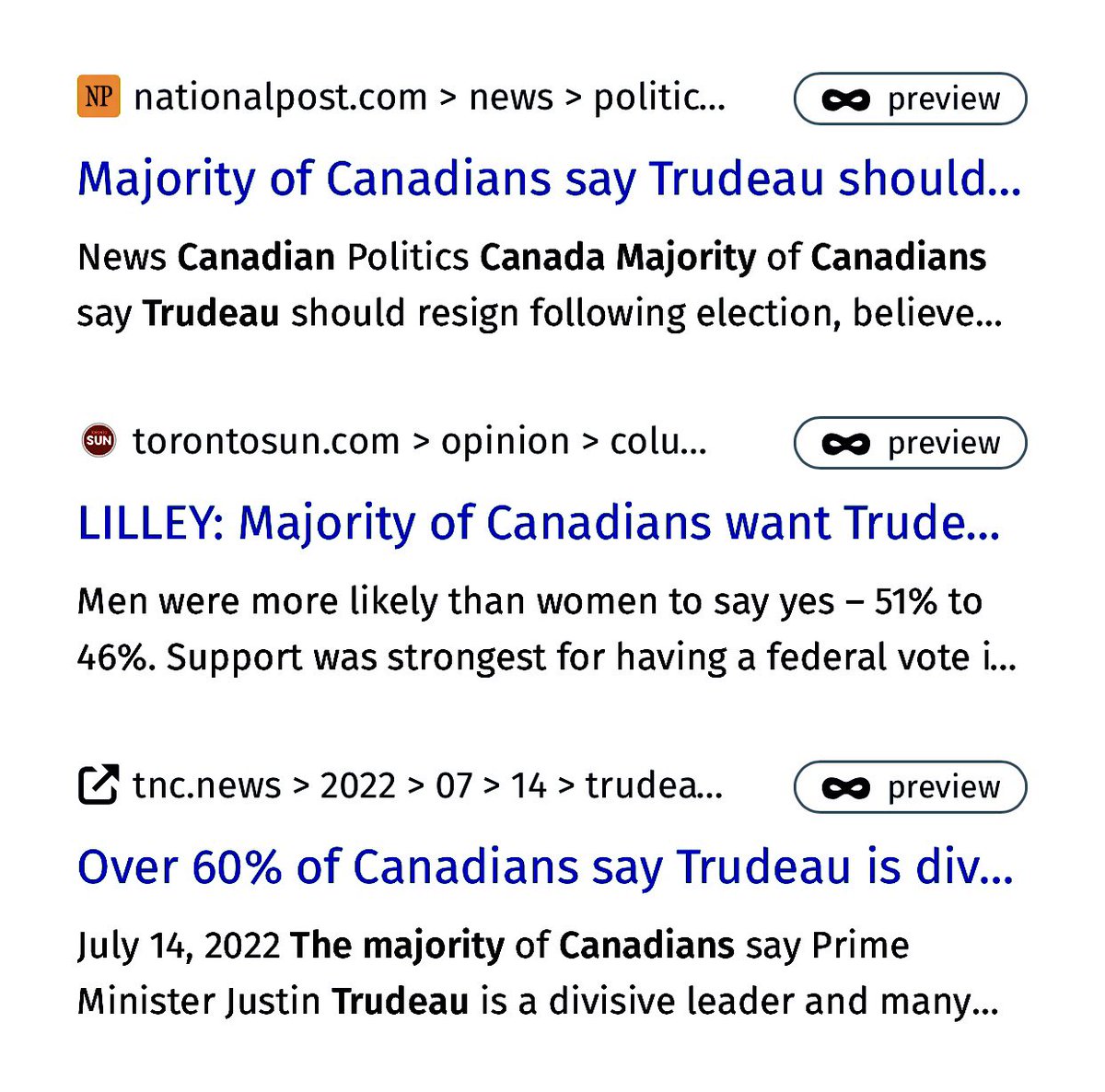The image is a screenshot displaying various search results related to Canadian politics. At the top left corner, there's a small orange square logo featuring the letters "NP," indicating it's from National Post. Adjacent to the logo, in black text, it reads "nationalpost.com news politics," though some of the text is truncated. To the right, there's a dark green outlined button featuring an infinity symbol and the word "Preview." The headline, in blue text, states, "Majority of Canadians say that Trudeau should..." 

Under that, smaller black text provides additional information: "news Canadian politics Canada majority of Canadians say Trudeau should resign following election, believe..." 

Further down, there's a red circular icon with white lettering "SUN," next to black text reading "torontosun.com opinion," which is also truncated. Next to this, on the right, is the same green "Preview" button. 

Beneath this, another blue headline says, "Lily majority of Canadians want Trude..." In smaller black text below it, it says, "men were more likely than women to say yes 51% to 46%. Support was strongest for having a federal vote i..."

At the bottom of the image, there’s an icon resembling three-fourths of a square with an arrow pointing out, next to black text "TNC news 2022 0714 Trudea..." and, to the right, the same green "Preview" button. Below this is blue text stating, "over 60% of Canadians say Trudeau is div..." In smaller black text below it reads, "July 14, 2022 the majority of Canadians say Prime Minister Justin Trudeau is a divisive leader and many..."